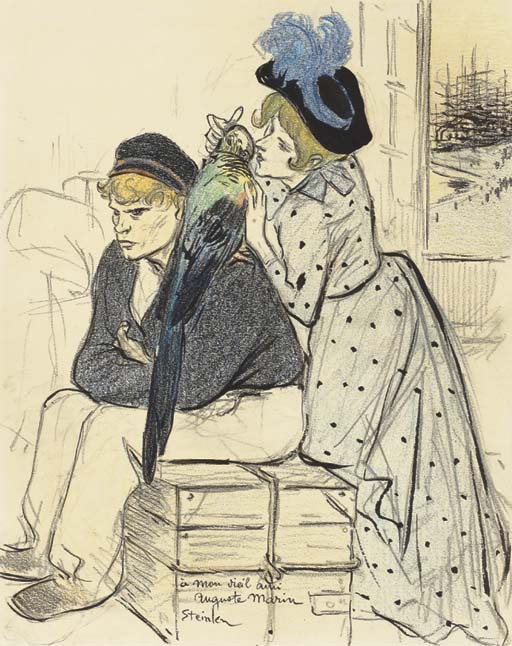The illustration, drawn on tanned paper with colored pencils or pastels, depicts a somber-looking dock worker from the 1800s. He is seated on a wooden crate tied with rope, wearing light-colored pants, dark shoes, a dark jacket over a white shirt, and a black sailor's cap over his curly blonde hair. A large blue and green parrot perches on his shoulder, facing away from him. The worker's arms are folded across his chest, and he leans slightly forward, appearing upset. Behind him, a woman with similarly golden hair, dressed in a light blue dress adorned with black polka dots, leans against his back. She sports a black hat with extravagant, billowing blue feathers and playfully interacts with the parrot, her face close to the bird. She has one knee resting on the crate. In the background, a window reveals a view of trees. The bottom center of the crate bears the artist's signature, which could be interpreted as "August Marin Steinem" or a similar name, although the exact letters are unclear.